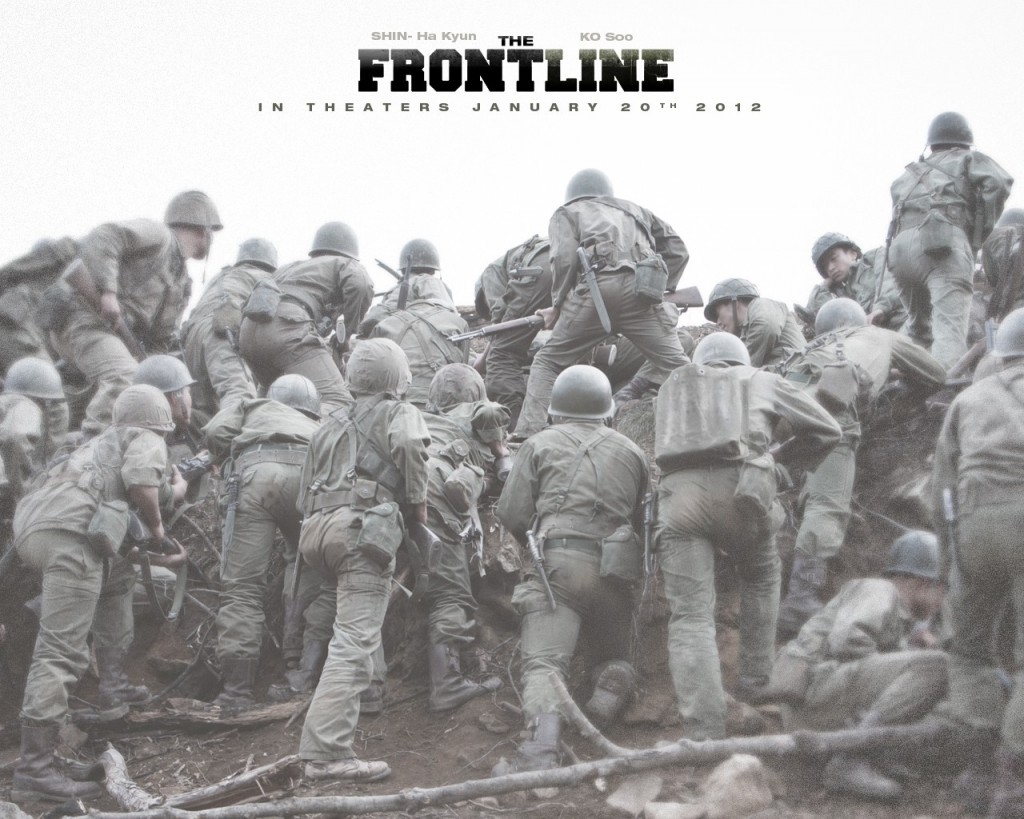The black-and-white photo depicts a group of soldiers facing away from the camera, suggesting a military conflict setting, possibly storming a beach or climbing a dirt embankment. The soldiers, wearing uniforms and hats, are captured in a moment of intense effort, appearing to either push against or scale a surface, with their guns held at the ready. The image features contrasting shades of green, brown, and gray, adding to a raw, gritty atmosphere. At the top center of the image, bold black text reads "The Front Line," followed by "In Theaters January 20th, 2012." Alongside this, the names "Shin Hakyeon" and "Ko So" are written in a lighter gray, hinting at prominent figures involved in the film. The overall composition suggests a dramatic scene set against a bare, rugged terrain, with branches and dirt accentuating the harsh conditions faced by the soldiers.